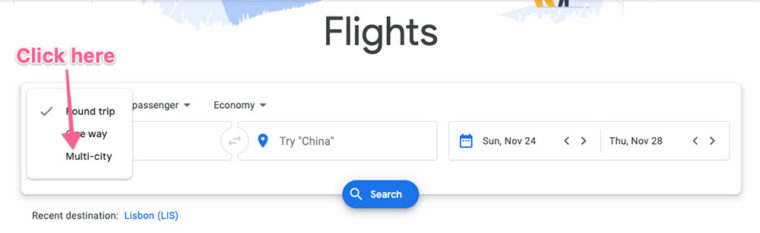The image header prominently displays the word "Flights" in black lettering against a predominantly white background, enhanced by subtle blue brush stroke accents. Below this, a light gray bordered text box is filled with multiple selection options. In the top section of this box, red text stating "click here" is accompanied by a downward arrow pointing towards the word "multi-city," which is integrated within a smaller white box alongside "round trip" and "one way" options.

Within the larger white rectangle, several input fields are clearly labeled. These include fields for "economy," "passenger," and "try China," the latter marked by a blue location pin. Adjacent, larger boxes are marked with specific dates: "Sunday, November 24th" displays a blue calendar icon, while the box next to it reads "Thursday, November 28th." At the bottom of this area, a blue oval button with the white word "search" invites user interaction.

In the lower-left corner of the image, the phrase "recent destinations" is noted in black text. Immediately following, "Lisbonne (L-I-S)" is listed in blue writing.